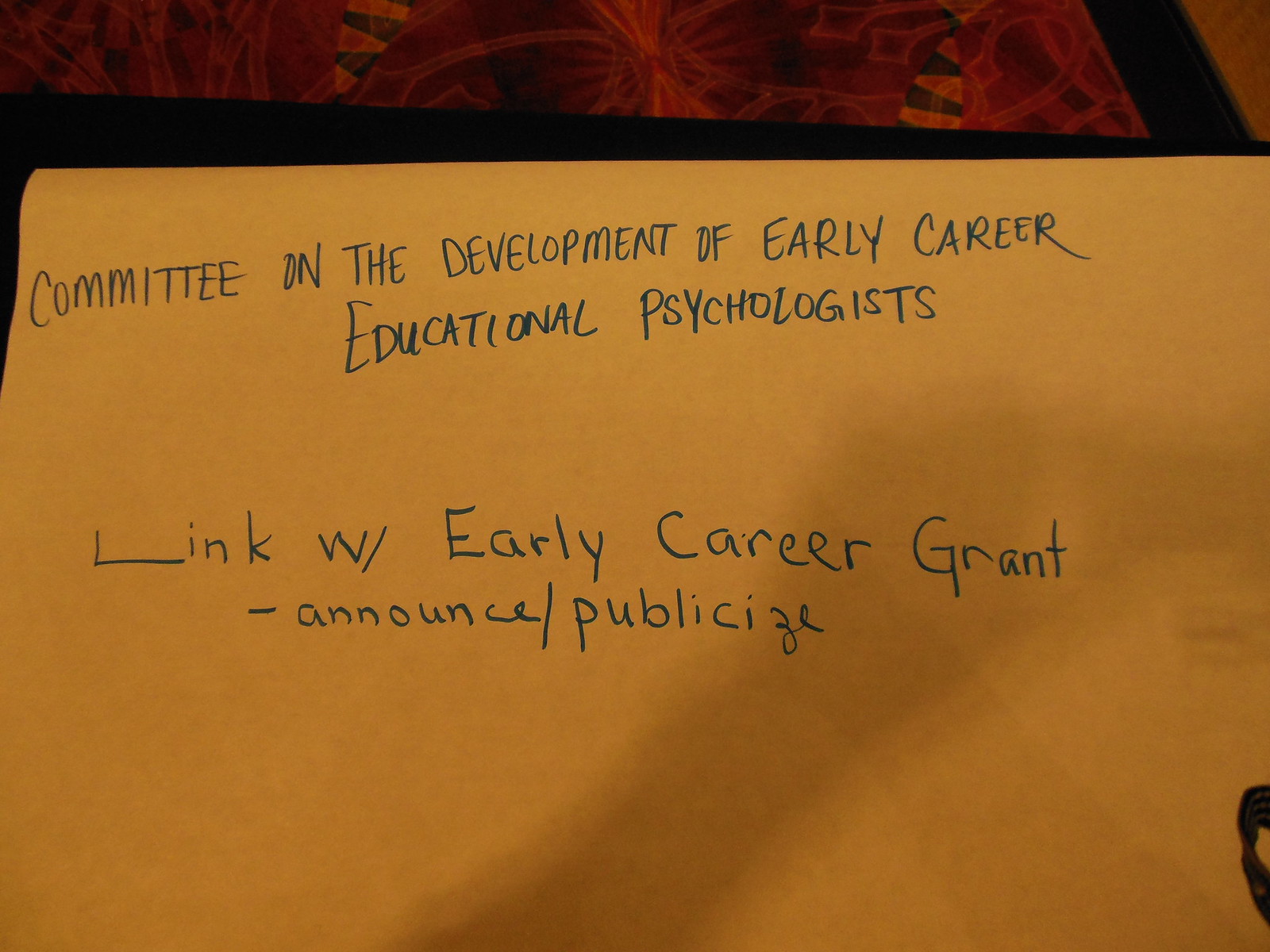This detailed caption combines and cleans up the various descriptions:

This photograph captures a handwritten note on a sheet of yellow paper, written in blue ink. The note is organized into two main sections, all in capital letters at the top: "COMMITTEE ON THE DEVELOPMENT OF EARLY CAREER EDUCATIONAL PSYCHOLOGISTS," followed by "Link with Early Career Grant," and then, "Announce/Publicize" in normal capitalization. Notably, the letter 'L' in "Link" is elongated, and "with" is abbreviated as "W/". The paper is placed on what seems to be a black object, potentially a folder or device, with an orange geometric design visible in the background, suggesting it might be laying on a patterned carpet or fancy surface, possibly at a convention. A shadow, presumably the photographer's hand holding a camera or smartphone, crosses the middle of the image, adding a candid element to the scene.